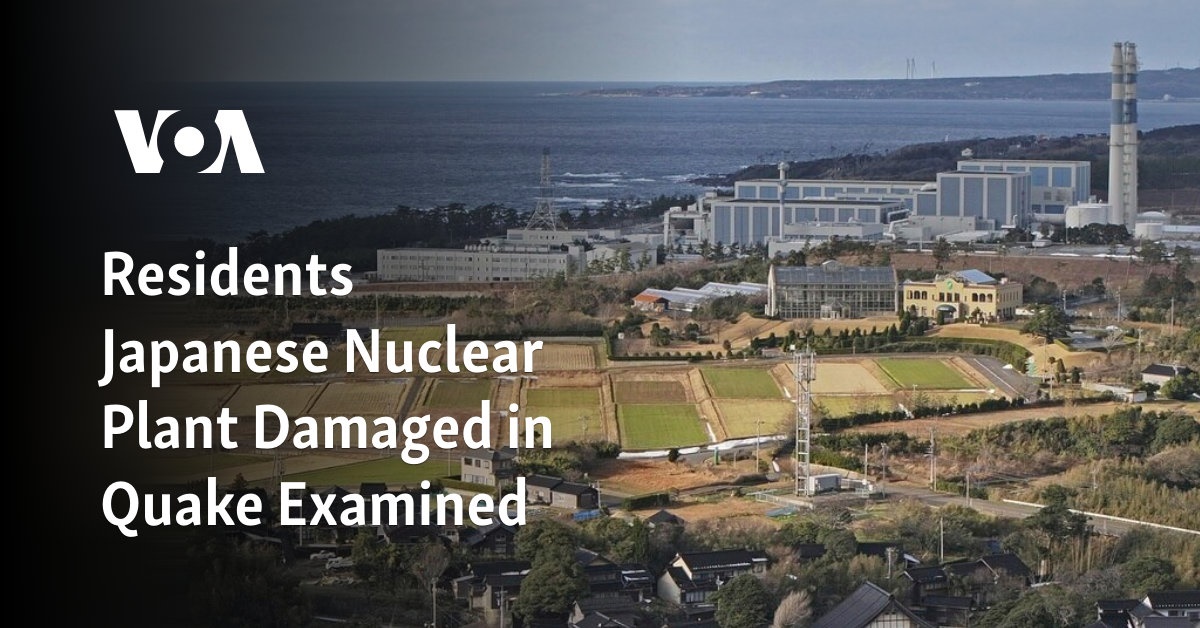This poster image appears to be a horizontal rectangle depicting an aerial view of a Japanese coastal area with a significant emphasis on a damaged nuclear plant. The prominent features include a large white "V" followed by a gray "O" with a white center, and a white "A" resembling an upside-down "V" on the top left corner, forming the acronym "VOA." The main headline in large white text reads: "Residents Japanese Nuclear Plant Damaged in Quake Examined."

In the background, extending across the entire top of the image, is a stretch of ocean with some distant land and a light gray sky. The top right of the image showcases a cluster of buildings, identified as a Japanese nuclear plant, which includes a tall tower structure. Below this area, there are various buildings and grassy areas interspersed with brown patches and brush, possibly indicative of recreational spaces or fields. The bottom middle section features several buildings that could be homes, surrounded by more vegetation.

To the left side, the water tinges a darker blue, blended with some white patches. The landscape reveals a mix of white, yellow, and glass buildings, some with distinct roof colors like blue and black. There are also fields displaying shades of white, green, tan, and gray interspersed among green trees and brush.

Overall, this image captures the complex landscape of Japan’s coastal area post-earthquake, highlighting both natural and man-made elements amidst the aftermath of a significant event.